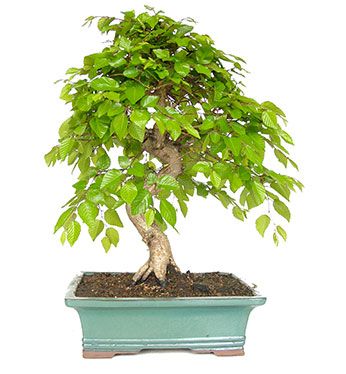The image depicts a potted plant against a stark white background, typically seen on product-selling websites. The planter is a rectangular, teal-colored clay pot with a slightly wider top than the base, and tiny quarter-inch legs at the bottom where no paint was applied. It's filled to the brim with soil. The plant itself resembles a small tree or bush with a light tan, zigzagging trunk that gives a snake-like appearance. Adorned with numerous small to medium-sized, bright green leaves, some with a yellowish tinge, the plant appears healthy and vibrant. The tree's leafy branches droop slightly, covering much of the tree and contributing to its lush appearance. The clean, white background suggests the image has either been digitally altered or shot in a controlled setting, making it difficult to discern the scale or context of the environment.